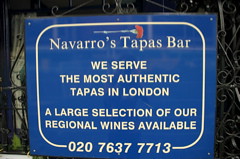The image captures a blue banner attached to a metallic fence, with a design that gives the impression of a window sign. The banner has a rounded white border framing the text, which reads: "Navarro's Tapas Bar" in standard font, followed by the phrases "We serve the most authentic tapas in London" and "A large selection of our regional wines available," both in capital block letters. At the bottom of the banner, also in white font, is the contact number: 020 7637 7713. The background outside the banner features dark, streaky reflections suggesting a glossy window surface behind the fence, providing a contrast to the vivid blue and white text of the sign. Additionally, there is a small flower-like design with a reddish top positioned above the establishment's name, adding a subtle decorative element to the banner's layout.